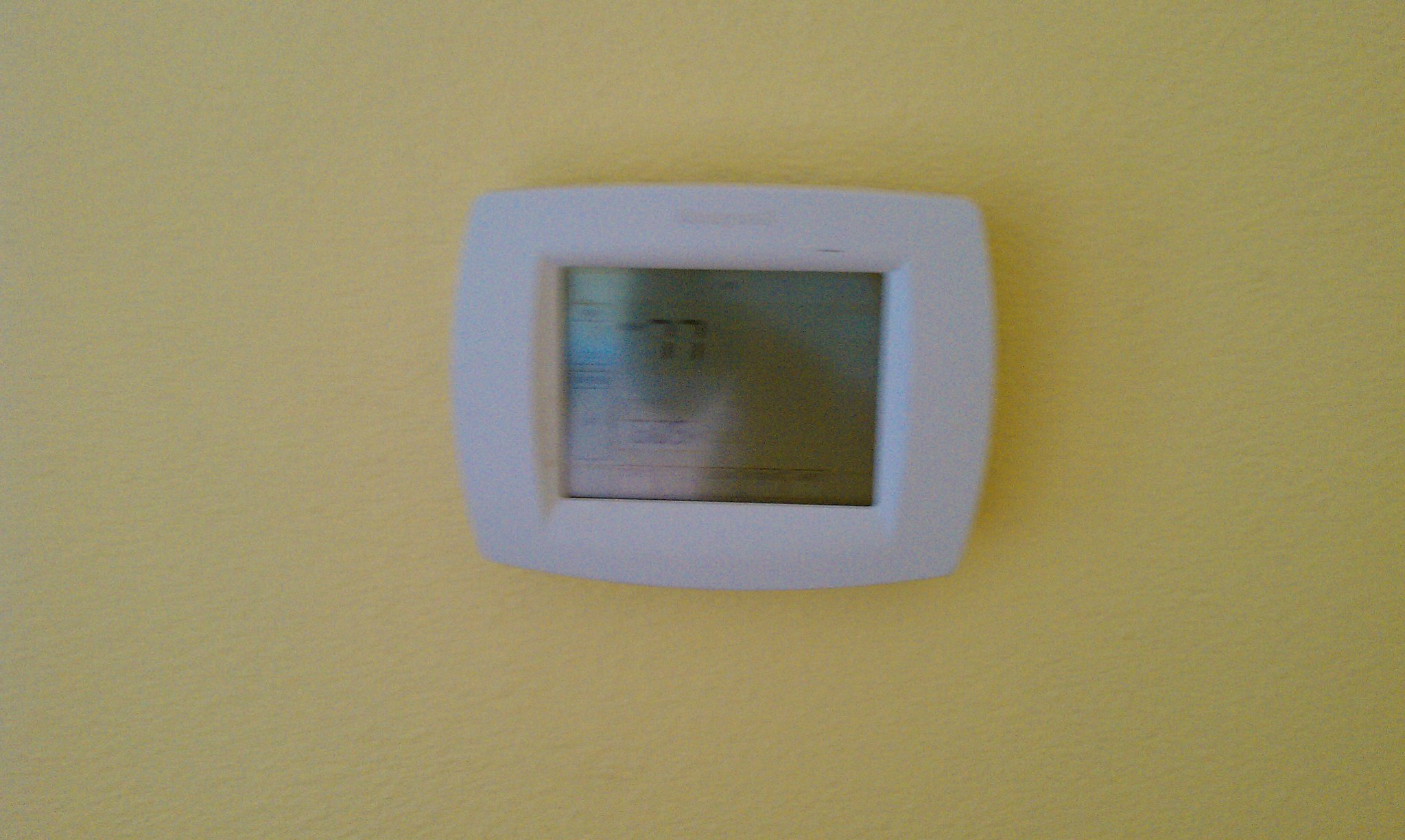A brightly painted yellow wall serves as the backdrop for a white rectangular thermostat, likely made of plastic. The texture of the wall adds to the aesthetic appeal of the scene. The thermostat features a dimmed LCD touchscreen, with partially visible text at the top that is unreadable. The display clearly shows a temperature of 77 degrees. There are additional boxed writings on both the left and right sides of the screen, though the dimness and shadows make them difficult to decipher. A shadow of a person standing in front of the thermostat is also cast on the wall, further obscuring any fine details. The overall image is somewhat shadowed, and the textured wall adds an additional layer of depth to the scene.